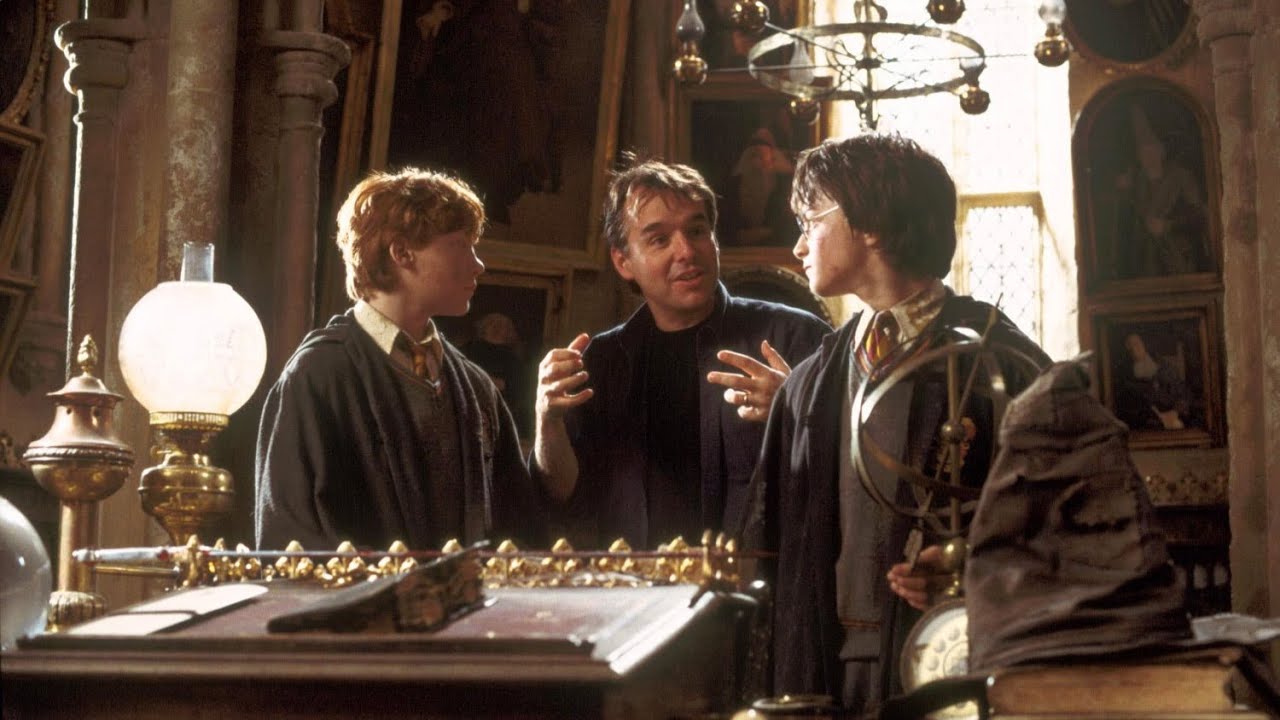In this detailed scene from a Harry Potter movie, we see Harry Potter alongside two other individuals inside a grand hall adorned with various items. Harry, positioned on the right, is intently examining a round device resembling a compass, its metal spokes gleaming. He wears a school uniform consisting of a blue coat, a white shirt, and a yellow tie. To his left, a man dressed in dark clothing, possibly a professor or mentor, gestures animatedly with his hands as he speaks to Harry. This man is flanked by another boy with orange hair—Ron Weasley—who also wears a similar school uniform and looks attentively at the gesturing man.

The setting is rich in detail: overhead, a large chandelier, silver in color, hangs majestically, casting a glow in the room. Directly behind the trio, a giant window lets in ample light, illuminating the scene. The left side of the image reveals a brightly lit lamp with a white bulb and a gold base. In front of them, a table cluttered with items like small metal figures, a silver chalice, and books—one partly open, another with an envelope on it—suggests a place rich in magical artifacts. There is also a dark-colored bag on the right countertop next to the books.

The ambient decor of the hall includes columns that lead to other areas, walls decorated with hanging items, and various golden accents catching the light. Collectively, the detailed attire of the characters and the intricate setting create a vivid snapshot of the magical world, accentuating the rich textures and atmospheric environment typical of a Harry Potter scene.